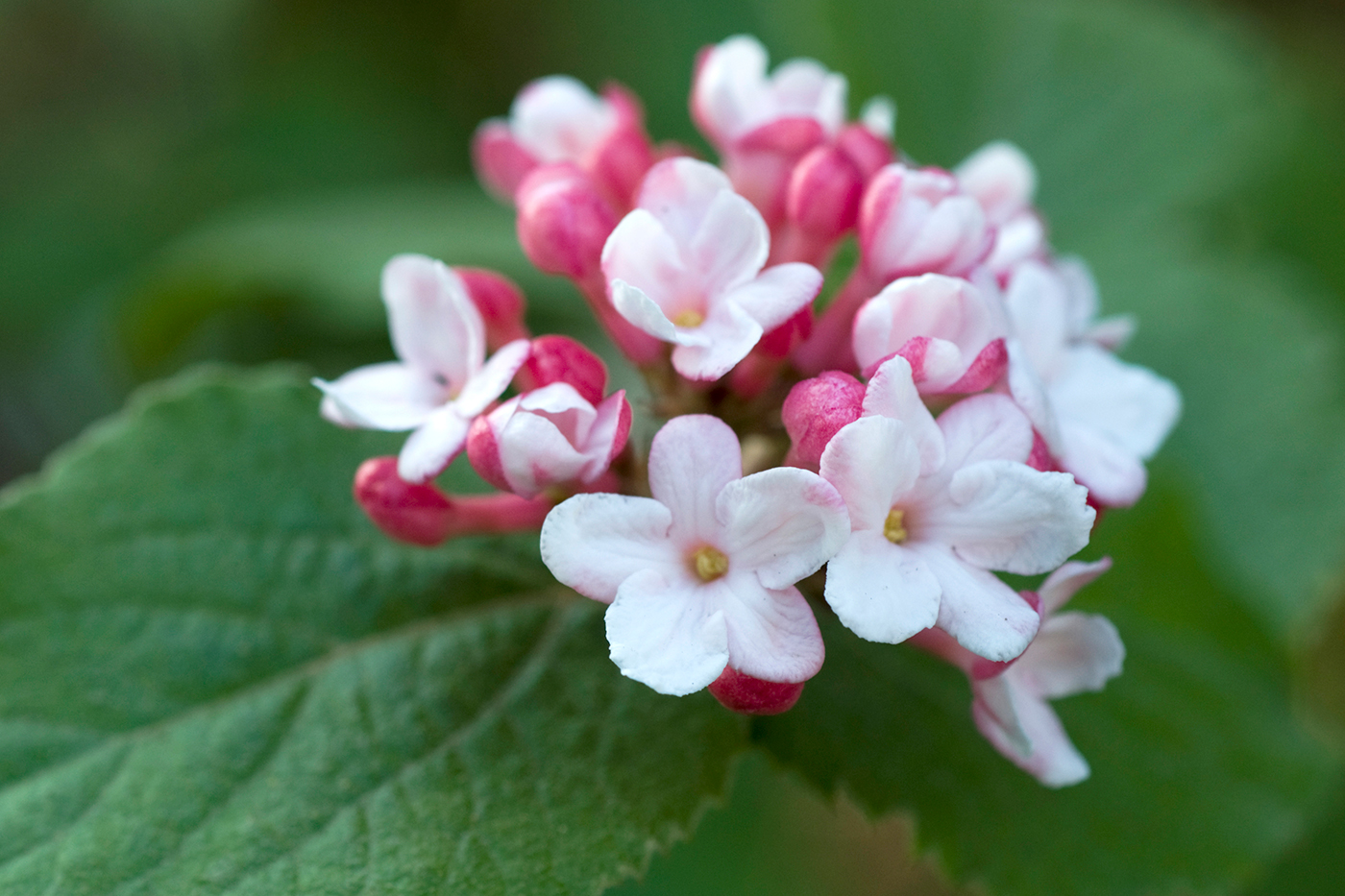This is a close-up photograph of a cluster of delicate flowers, resembling a hyacinth, in various stages of bloom. Positioned at the center of the image, the flowers exhibit a graceful spectrum of white petals with pinkish edges and a small yellow dot of pollen in the middle of each. The scene features about a dozen flowers, with five fully bloomed, displaying their five extended petals, and numerous unopened pink buds. The flowers range from fully open to semi-open and partially blooming, creating a dynamic display of growth.

The vivid green leaves serve as the backdrop, accentuating the flowers' colors. One prominently detailed leaf is visible in the foreground, showing intricate veins and texture. The rest of the leaves and background are blurred, creating a soft focus that draws attention to the centrally located flowers. Despite the blur, the vibrant greenery and the sharp focus on the foreground flowers combine to provide a striking contrast. The overall lighting ensures that the colors, while vivid, are not overly bright, maintaining a natural and refreshing ambiance.